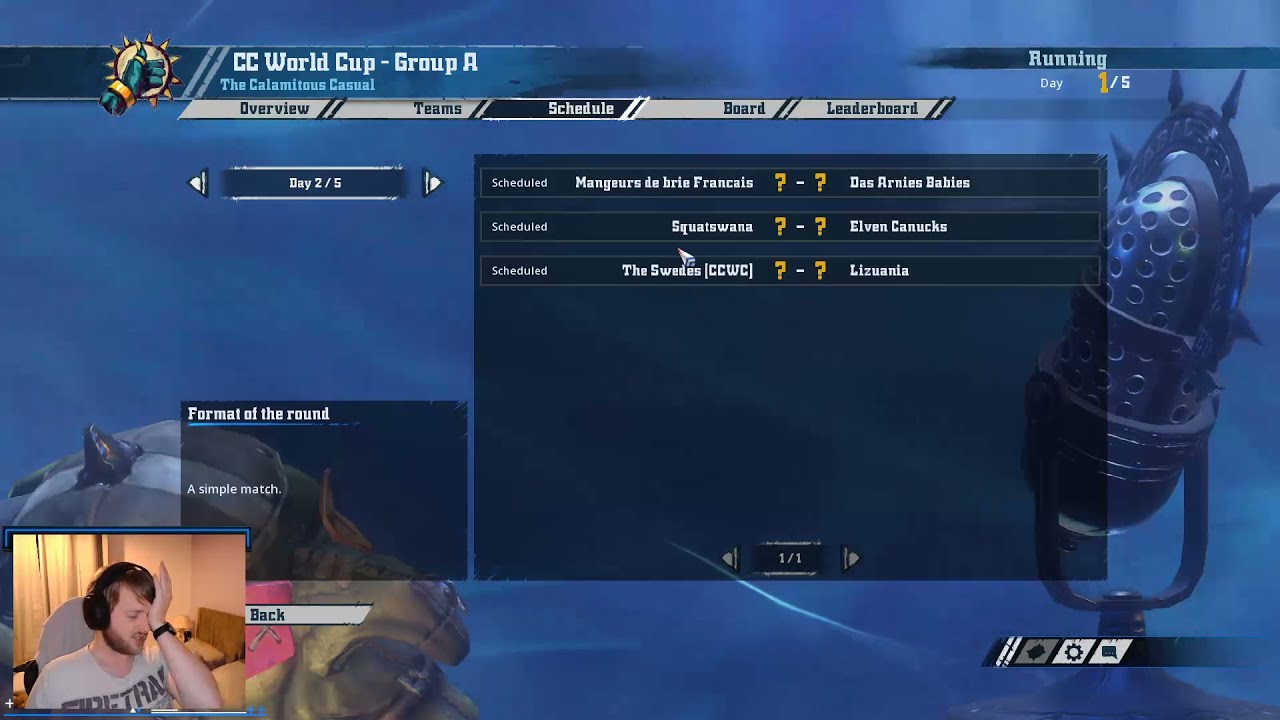The image is a detailed screenshot of a streaming session where a man is broadcasting himself playing what appears to be an RPG or MMORPG. Displayed on the computer screen is a blue-background interface titled "CC World Cup Group A" at the top left and showing it is Day 2 of 5 in the event. The interface features tabs labeled "Overview," "Team," "Schedule," "Board," and "Leaderboard," with the "Schedule" tab currently selected. Various player names in French are listed, but many match details are indicated with question marks. The upper right corner of the screen prominently shows the status "Running," suggesting ongoing gameplay.

The lower left corner of the game interface includes a live feed of the streamer, a white man with brown hair and a brown beard, wearing a gray shirt with text, and black headphones. He is seen sitting in a white chair, holding his hand to his face in a classic face-palm gesture, appearing visibly frustrated or disappointed. Behind him, the background of his room is visible.

A notable background detail in the screenshot includes a metallic object resembling an old cardio microphone or perhaps a bell, adorned with decorative metal spikes, positioned on the left side of the image. Additionally, there seems to be the figure of a green goblin-like character in the lower part of the screen amidst the gaming interface, adding to the overall theme and ambiance of the game.